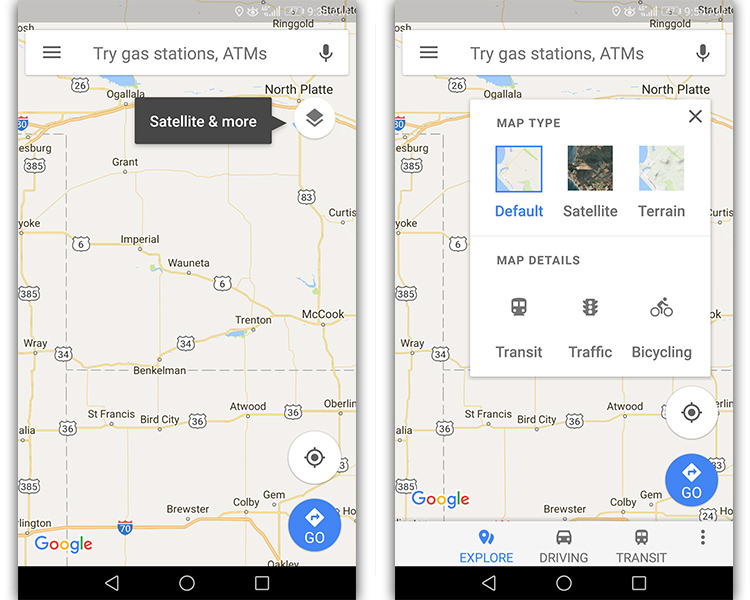The image consists of two side-by-side smartphone screenshots displaying a navigation app. Both screenshots feature a brown status bar at the top, revealing incomplete details about battery life and signal reception. Below this, a white search bar stretches across both screens, marked with three horizontal lines on the left and a microphone icon on the right. The search bar contains the text, "Try Gas Stations, ATMs."

The left screenshot showcases a detailed map rendered in tan, accented by blue bodies of water and yellow roads. Notable cities such as Grant, Imperial, St. Francis, Bird City, Atwood, McCook, and Brewster are highlighted. Key routes identified on the map include Route 385, Route 6, Route 34, and Route 36. At the map's upper section, a black rectangle displays the options "Satellite" and "More," accompanied by a diamond symbol and a white circle. Near the bottom right corner, there is a white circle containing a directional icon, and a blue circle labeled "GO." At the very bottom, the "Google" logo is displayed, beneath which lies a black line featuring a back button, a home button, and a square button for recent apps.

The right screenshot presents a zoomed-in version of the same map area under the same white search bar. Superimposed is a large white rectangle titled "Map Type," featuring three different map options: Default, Satellite, and Terrain, each represented by a respective thumbnail. Below these, "Map Details" are listed with icons for "Transit" (a bus), "Traffic" (a traffic light), and "Bicycling" (a bicycle), indicating optional map overlays for various travel details.